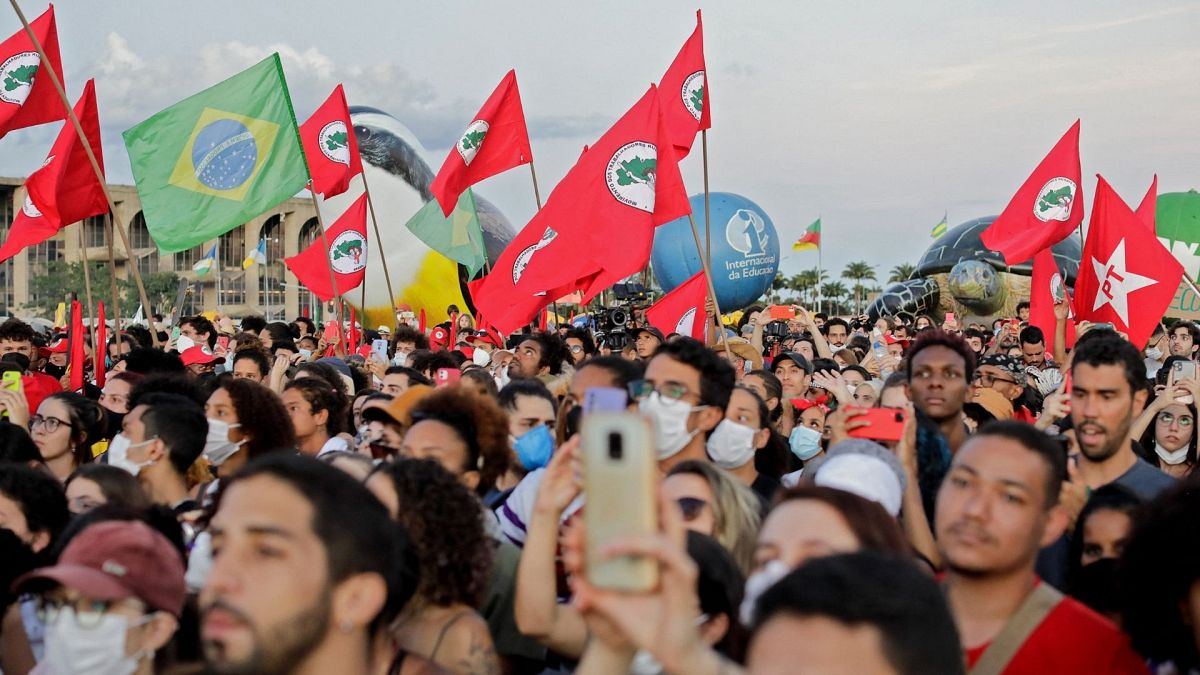The image captures a densely packed outdoor crowd, potentially a protest or a rally, with many young attendees. The crowd is holding a mix of flags, prominently featuring the Brazilian flag and numerous red flags adorned with white circles in the center. The scene is vibrant with a palette of colors including red, green, white, blue, and yellow. Numerous participants are wearing surgical masks, suggesting it might be during, or shortly after, the COVID pandemic. Several people are raising their phones, presumably capturing photos or videos. In the background, there's a notable sculpture of a tortoise and other inflatable figures like a penguin and a blue balloon with an eye. The backdrop includes what appears to be a government building, which adds to the sense of an organized event. A man dressed in red, carrying a pack with canvas straps, is seen looking directly at the camera, adding a personal touch to the bustling scene. The visible text, "international de educado," hints at an educational or international focus of the gathering.